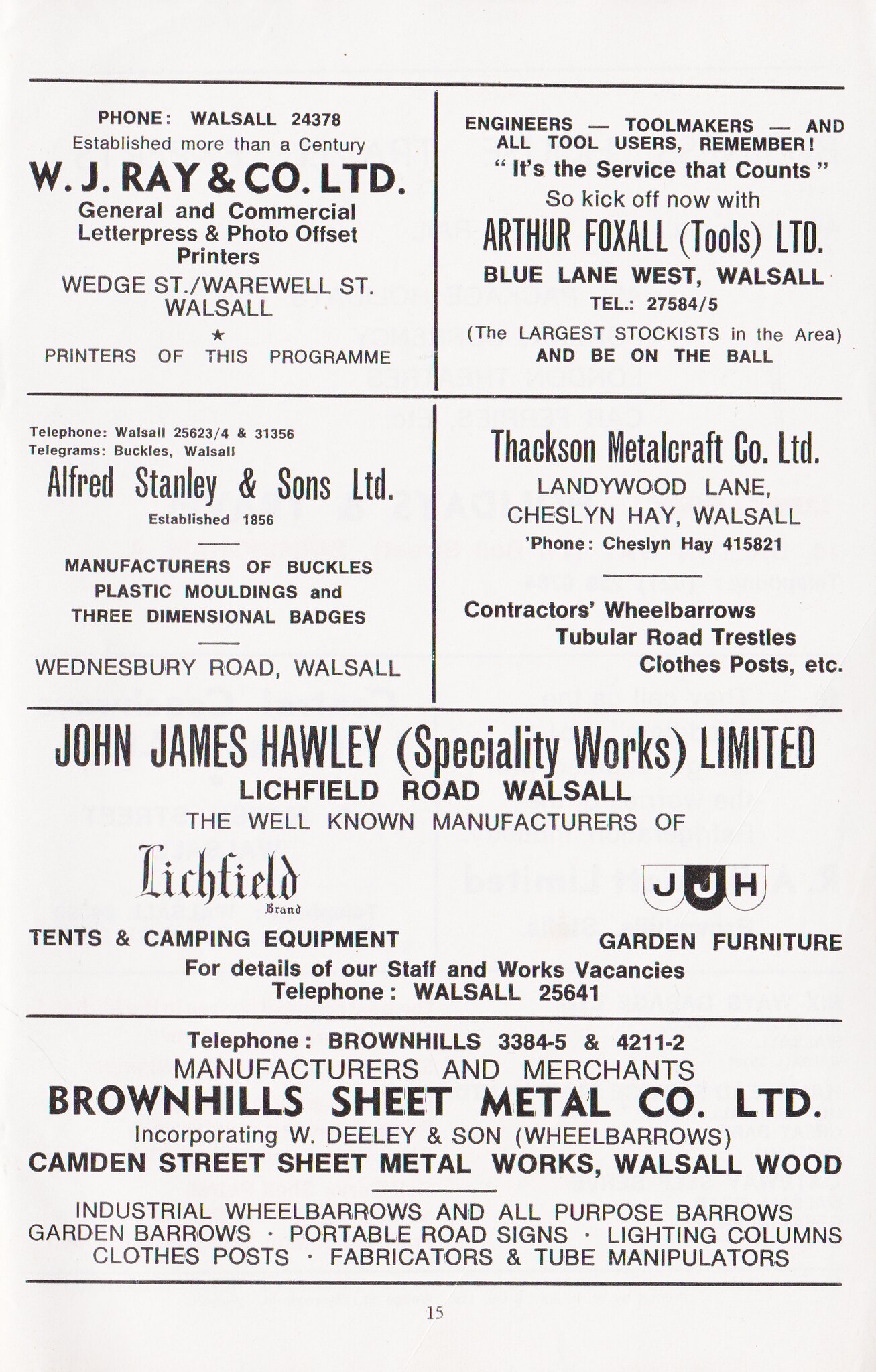This black and white image depicts a page of advertisements that likely originates from an event program. The layout consists of a two-by-two grid on the top half, featuring four distinct advertisements, each separated by black dividing lines, while the bottom half comprises two larger horizontal advertisements, also divided by similar lines.

At the very top left, there is an ad for W. J. Wray & Co. Ltd., general and commercial letterpress photo offset printers based at Wedge Street, Warewell Street, Walsall, also noted as the printers of the program. Adjacent to it, in the top-right box, Arthur Foxall Tools Ltd. promotes its extensive stock of tools at Blue Lane West, Walsall. Below, on the bottom-left of the grid, Alfred Stanley & Sons Ltd., established in 1856 and located on Winnisbury Road, Walsall, advertises its production of buckles, plastic moldings, and three-dimensional badges. The final smaller ad in the top grid is for Thackson Metal Craft Co. Ltd., based at Landywood Lane, Cheslin Hay, Walsall, offering contractors' supplies like wheelbarrows and tubular road trestles.

The bottom half features two larger ads: on the left, John James Howley Specialty Works Ltd., known for the Litchfield brand tents and camping equipment, based on Litchfield Road, Walsall, provides details on their products and staff vacancies; on the right, Brownhills Sheet Metal Co. Ltd., incorporating W. Dealey and Son Wheelbarrows at Camden Street Sheet Metal Works, Walsall Wood, highlights their range of industrial wheelbarrows, garden barrels, portable road signs, lighting columns, and fabricators and tube manipulators. This detailed collage of advertisements showcases a variety of local businesses and products, all meticulously laid out on the page.